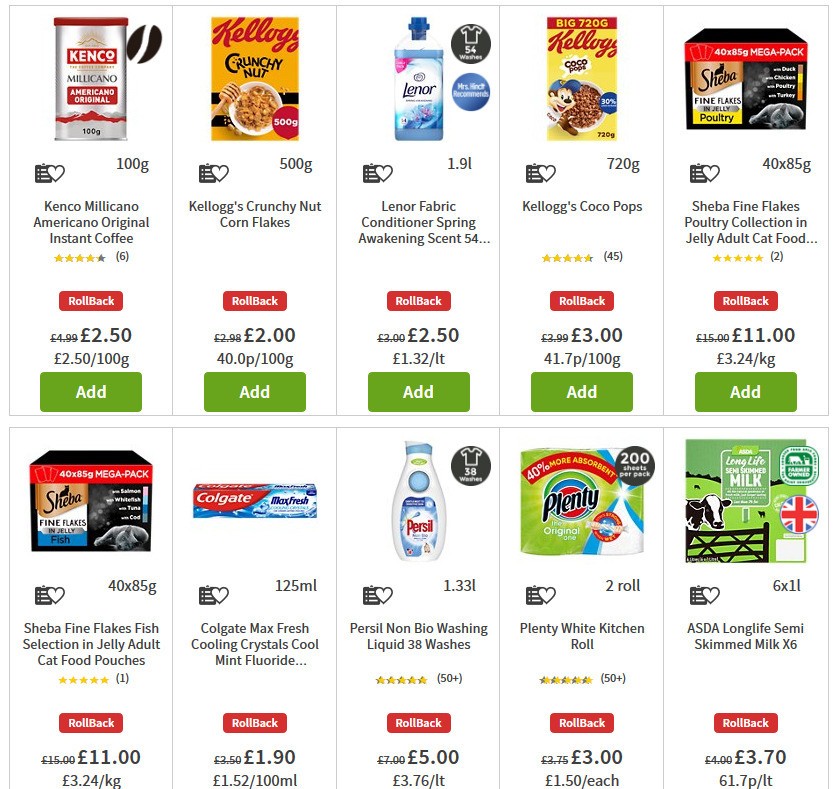The image, set against a white background, features several grocery store items with pricing and product information. At the top, a silver and red container labeled "Kinko Milicano Americano Original Instant Coffee" is featured, marked as a rollback price of £2.50 per 100 grams. A green "Add" button is visible next to this item.

Below this, a yellow and red box containing a honey spoon and a bowl of cereal is visible. The box is labeled "Kellogg's Crunchy Nut Cornflakes," priced at £2.40 per 100 grams.

Next, a bottle filled with blue liquid is labeled "Lenore Fabric Conditioner - Spring Awakening Scent." It is priced at £2.50 for a 1.32-liter bottle, equating to approximately £1.32 per liter.

Further down, another yellow and red box labeled "Kellogg's Cocoa Puffs" is visible, priced at £3.00 for 41.7 grams per 100 grams.

Lastly, some cat food is also present in the image, though further details are not specified.